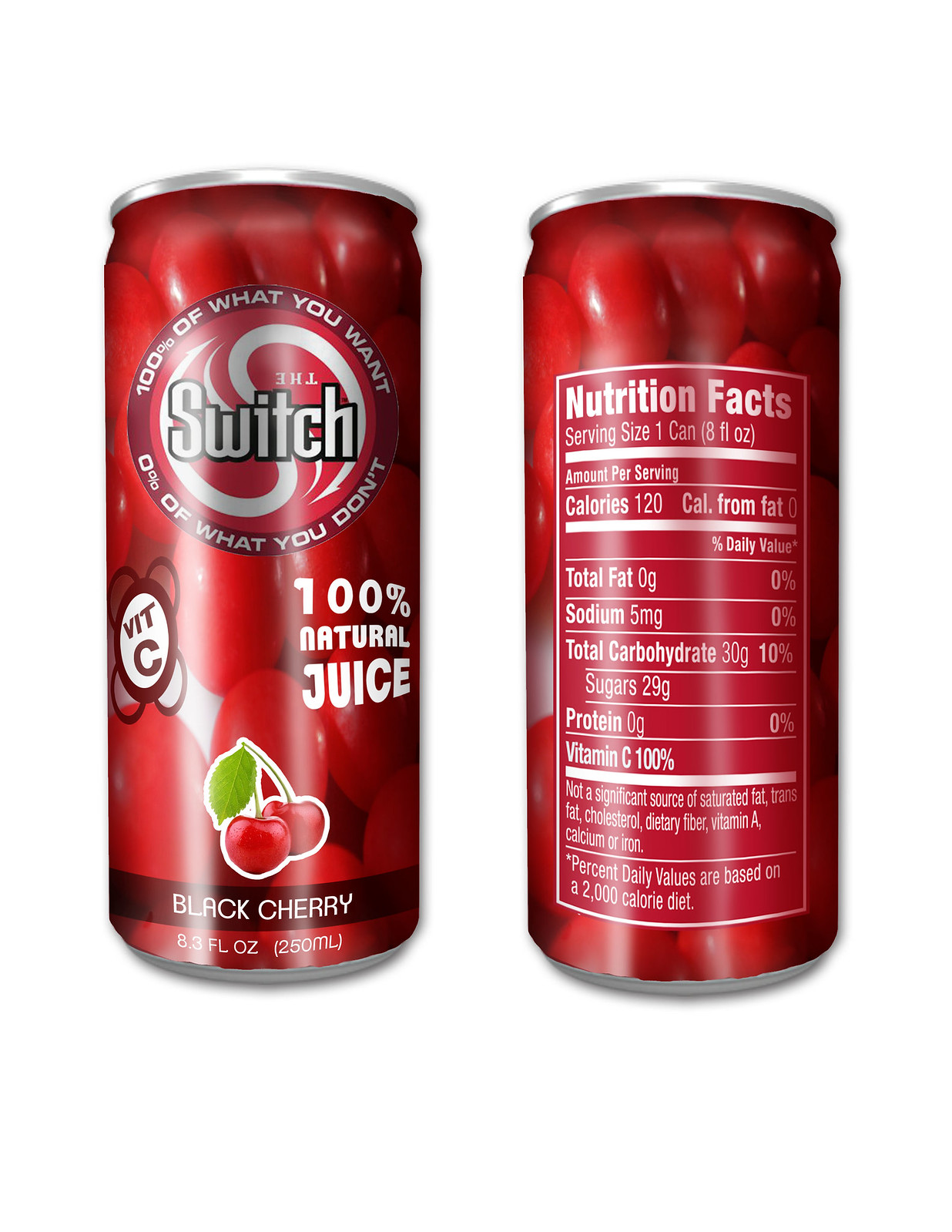The image showcases both the front and back views of an 8.3 fluid-ounce can of black cherry juice by the brand Switch. The can, which is tall and slender, stands against a white background, accentuating its vibrant red color. The front is adorned with images of juicy black cherries and text in white letters reading "Black Cherry" on a black cherry border. The phrases "100% natural juice" and "Vitamin C" are also prominently displayed in white. The Switch logo features an upside-down 'B' that forms part of a 'no reverse' symbol, embodying the slogan: "100% of what you want, 0% of what you don't." Turning to the back, the nutritional facts reveal that the serving size is one can (8.3 fluid ounces), containing 120 calories. The can emphasizes its natural ingredients with minimal components, highlighting its carbohydrate content.